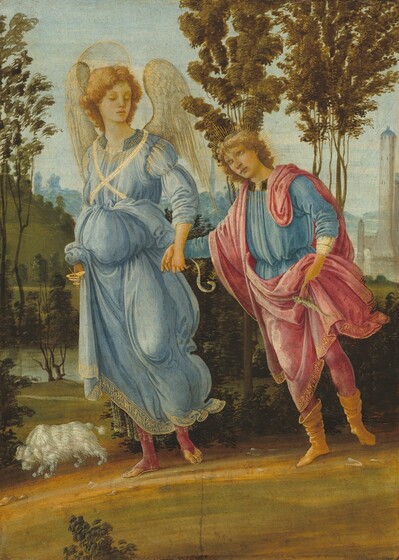This detailed painting depicts two figures standing on a streaked green and brown grassy surface. The figure on the left is a tall woman with short reddish-golden hair, dressed in a flowing light blue dress. She has distinct white angel wings emerging from her back and a faint white halo above her head. Her feet, adorned in pink covers, reveal her toes, and she gazes down and to the right.

The shorter figure, who reaches about shoulder height of the angel, stands to her right. This individual is attired in a blue tunic with white crests on the sleeves, complemented by a pink robe draped over the right side and cascading over the left shoulder. He wears white stockings and golden pointed boots, and his blonde hair frames his face as he looks up and to the left at the angel while holding her hand.

In the background, a picturesque wooden scenery is visible, featuring a tall, white tower with a blue rounded roof on the far right. Adding to the serene setting, a small body of water can be partially seen. To the left of the angel, a tiny white sheep with its nose to the ground and a puffy white tail positioned to the right enhances the pastoral atmosphere.